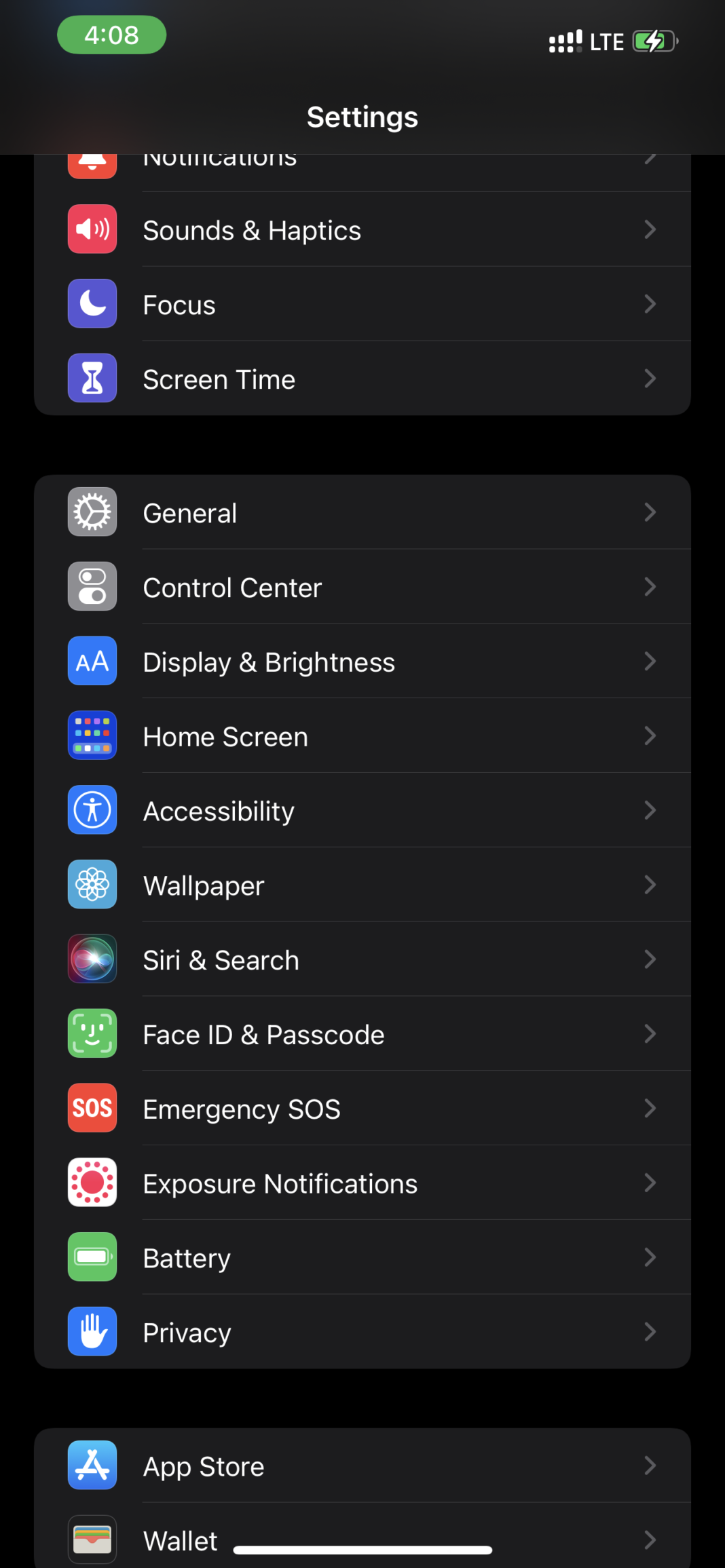This image is a cropped and enlarged screenshot of an iPhone's settings tab, displayed in Night Mode, indicated by the black background. In the top left corner, the time is encircled in green, signifying the user is currently on a phone call. The word "Settings" is prominently displayed in large white letters at the center top of the screen. The screenshot captures the middle section of the settings menu — the upper portion is partially cut off, but "Notifications" is still partially visible. The visible settings list includes "Sounds & Haptics," "Focus," "Screen Time," "General," "Control Center," "Display & Brightness," "Home Screen," "Accessibility," "Wallpaper," "Siri & Search," "Face ID & Passcode," "Emergency SOS," "Exposure Notifications," "Battery," and "Privacy." In the subsequent column, the "App Store" and "Wallet" options can be seen before being cut off. Each of these settings categories includes an arrow pointing to the right for further adjustment options.